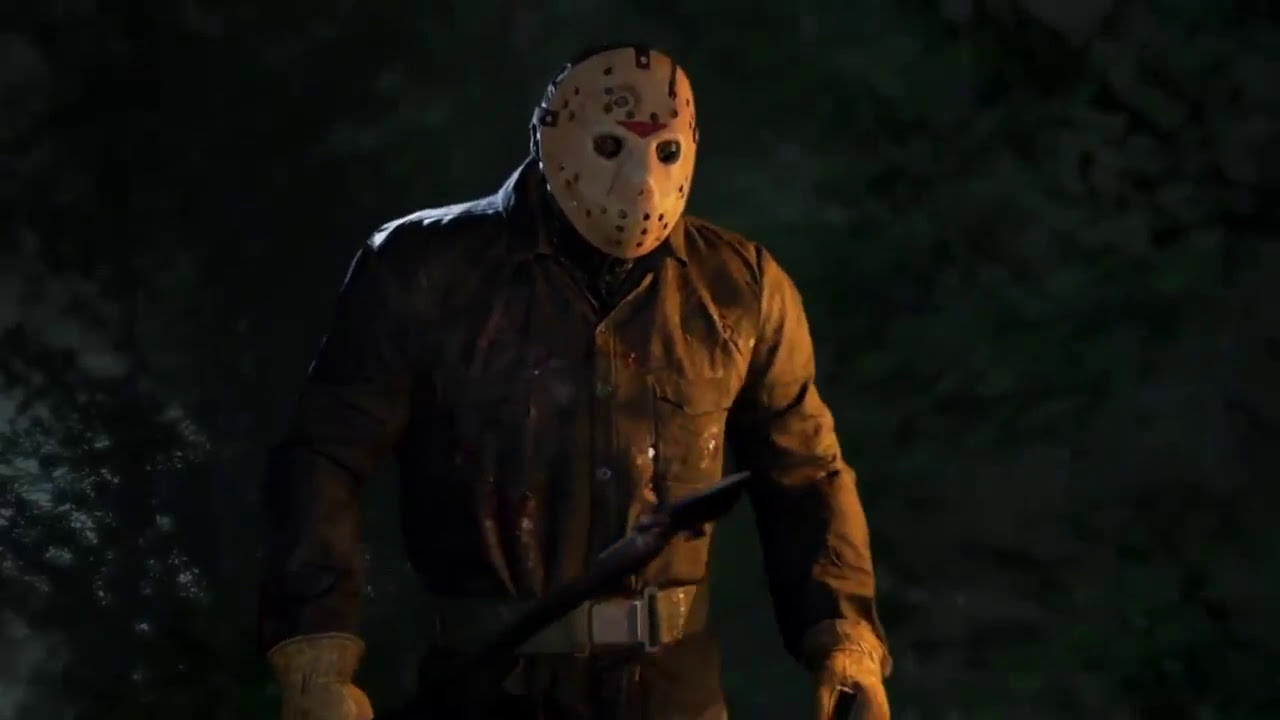The image is a still photo from a movie, featuring a nighttime scene with dark foliage in the background. At the center stands a large, ominous figure, clad in a stained and damaged white hockey mask with a downward-facing red arrow on the forehead. His eyes gleam from behind the mask's eye holes, and the mask also has holes near the mouth and is molded to include a nose. He wears a mechanic-stamped jumpsuit along with a utility belt around his waist, and mechanic's gloves cover his hands. In his right hand, he holds a wrought iron fire poker. The details of his attire include a heavy gray shirt that complements his menacing presence. There is a hint of a bladed weapon or item with a grayish tip that appears to be stabbed into his chest, adding to the overall eeriness. The background also features some black rocks in the lower-left corner, while the rest is consumed by dark shadows. The image is devoid of text or additional objects, measuring approximately 7 inches wide by 5 inches tall.